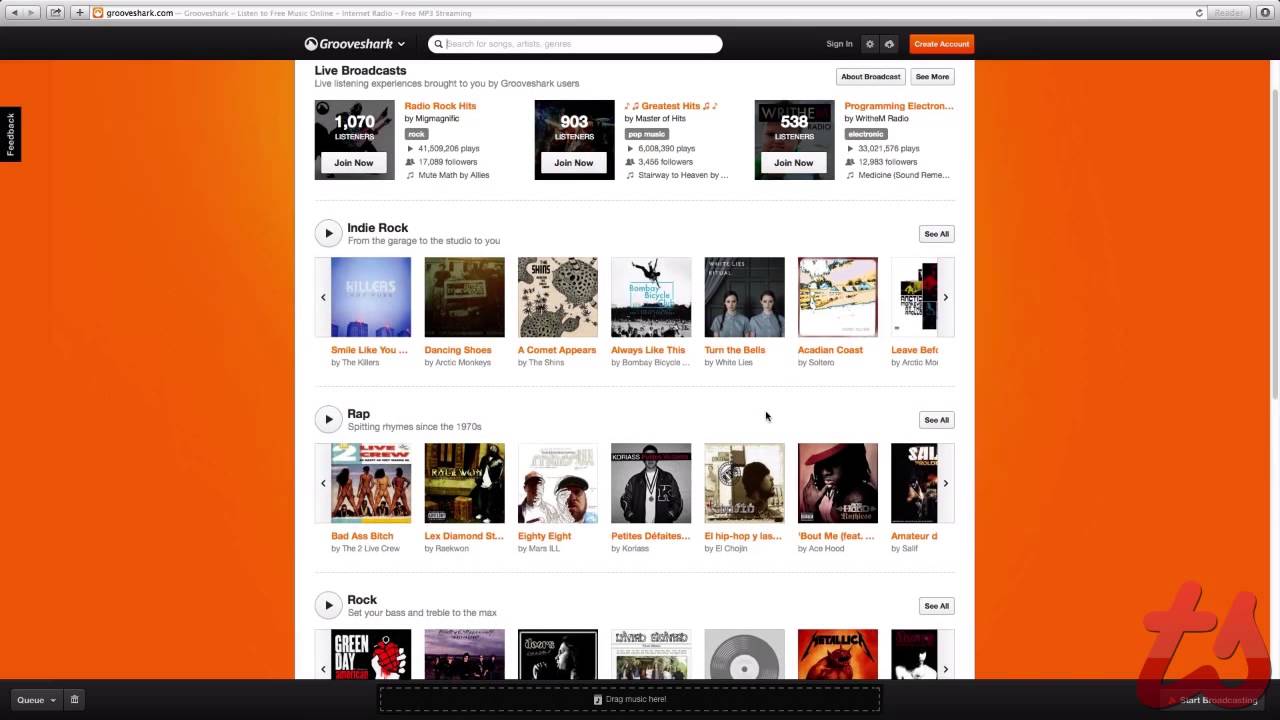The image features a vibrant orange background with a prominent search bar at the top. Below it, an orange rectangle with white text reads "Create Account," while a black rectangle with white text reads "Sign In." The layout suggests a live broadcast interface showcasing three images. A section labeled "Suspensions" appears to be brought to the viewer by a group link, possibly involving users, with a theme of Indie Rock prominently featured.

The screen is populated with numerous images related to music, including both pictures and videos that might represent songs. A specific section highlights rap music with corresponding images and videos. In the same area, a black cursor is visible, indicating user interaction.

Additionally, a gray rectangle containing the text "See All" in black appears in both the first and third sections of the interface. The third section also features a selection focused on rock music with several associated pictures.